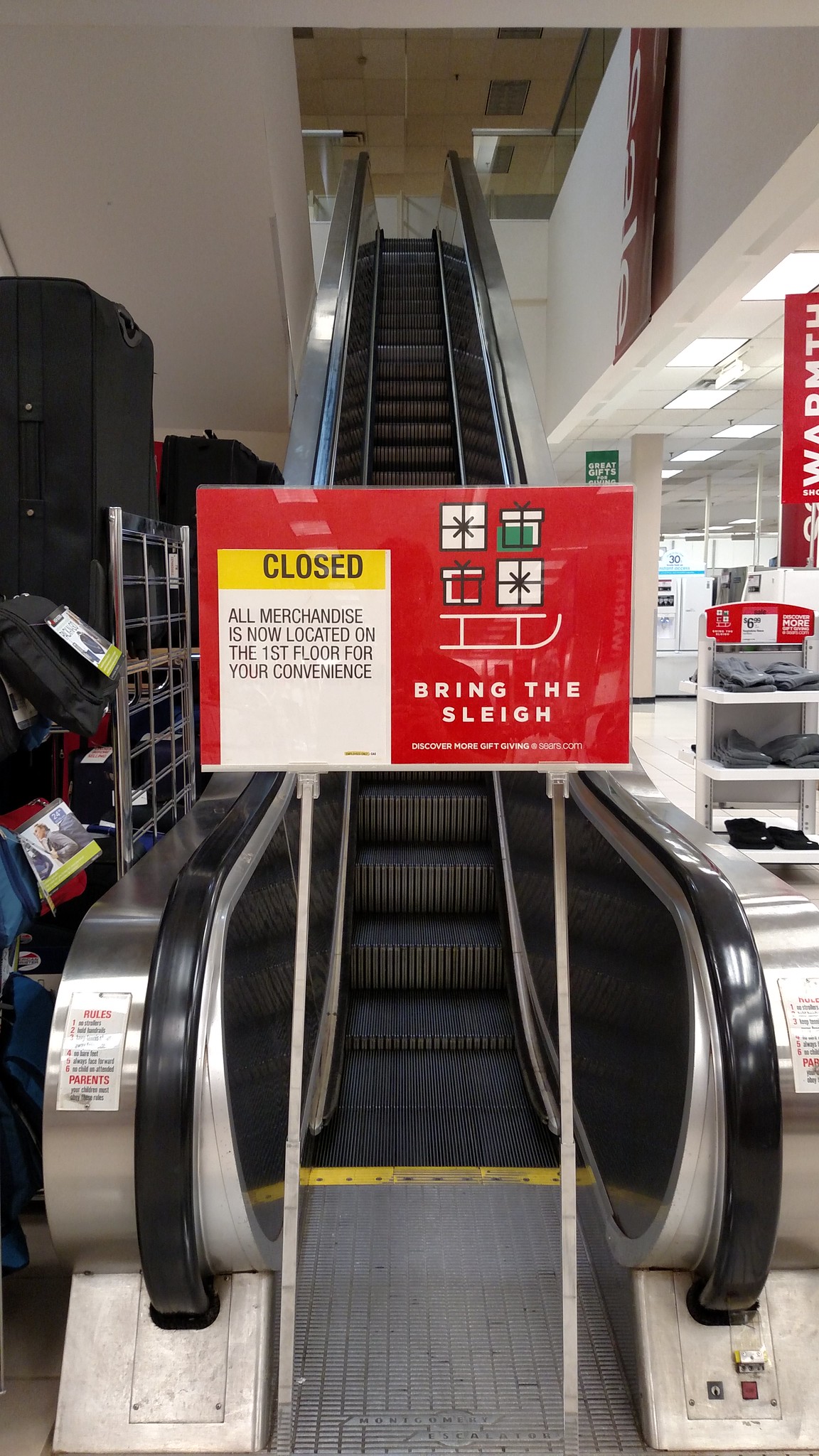This photograph captures a department store escalator out of service. A prominent red "closed" sign, with the message "All merchandise is now located on the first floor for your convenience," is placed in front of the escalator. The sign features a festive Christmas slogan, "Bring the Sleigh," adorned with a simple white line drawing of a sleigh and four wrapped gifts, showing the tops of two and the sides of the other two.

To the right of the escalator is a shelving display. To the left, a metal rack showcases an assortment of luggage, including backpacks and large suitcases. The metal rack is designed like a square fence, although the image only reveals its front side. In the background, a section of the store can be seen, though the signage in this area is indistinct.

Fluorescent lights illuminate the first floor of the store, casting a bright and functional ambiance. The overall scene underscores the closed status of the escalator, redirecting customers to explore merchandise conveniently located on the first floor.